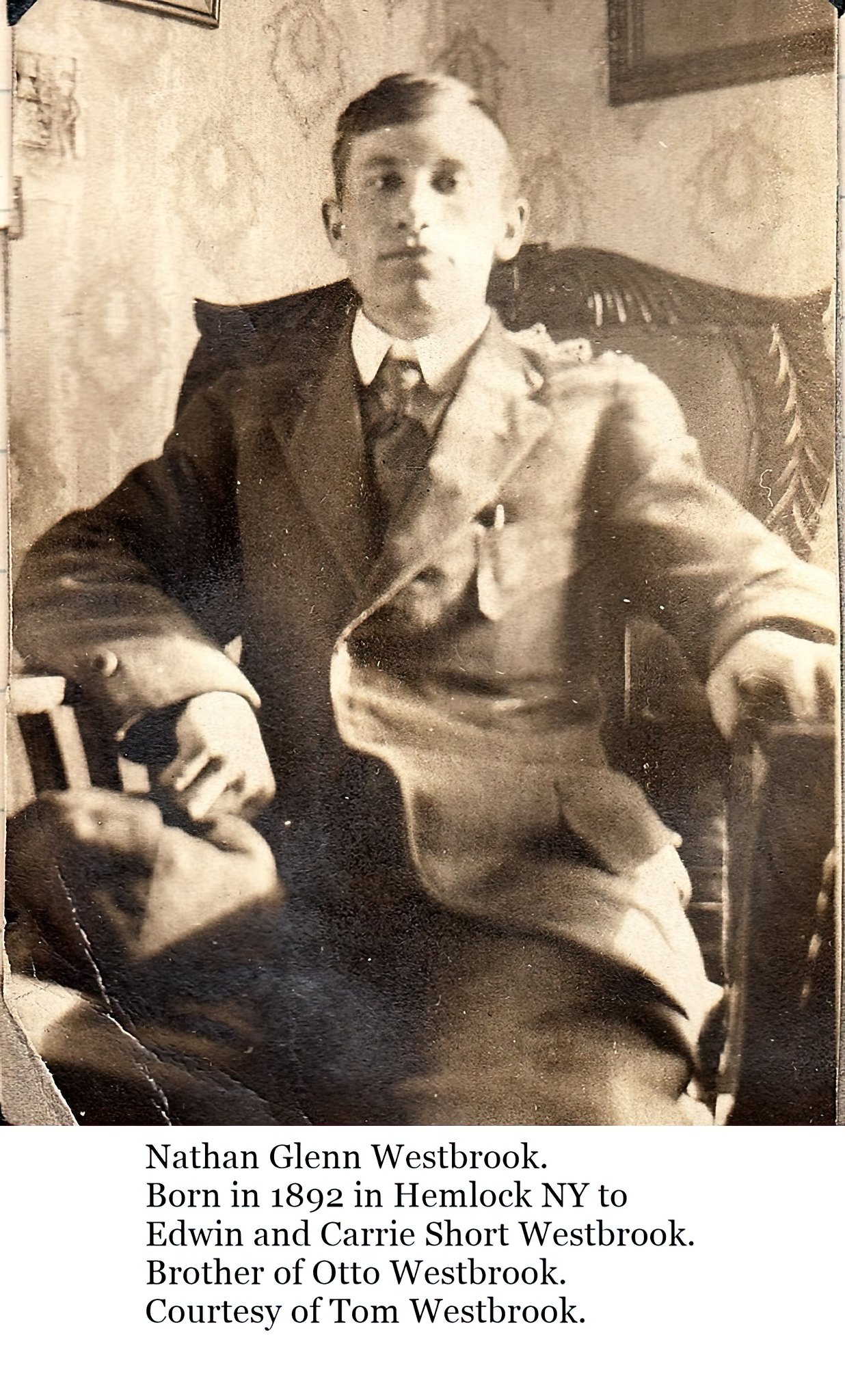The image is a sepia-toned, black-and-white photograph of a young man named Nathan Glenn Westbrook, born in 1892 in Hemlock, New York, to Edwin and Carrie Short Westbrook. He has a brother named Otto Westbrook, and the photo is courtesy of Tom Westbrook. Nathan, dressed in a buttoned-up dress suit with a lapel and a high-collared white shirt adorned with a tie, is sitting in a high-backed wooden chair with leaf flourishes around the cushion. His short brown hair is neatly swept to the side, and he gazes directly into the camera with a serious expression. His arms rest on the armrests of the chair; his right elbow is on the armrest with his hand toward his leg, possibly holding a bag or hat, while his left hand grips the edge of the armrest. The backdrop of the photo features patterned wallpaper and two picture frames. The detailed woodgrain and ridges of the chair are visible, adding depth to the indoor setting of the photograph.